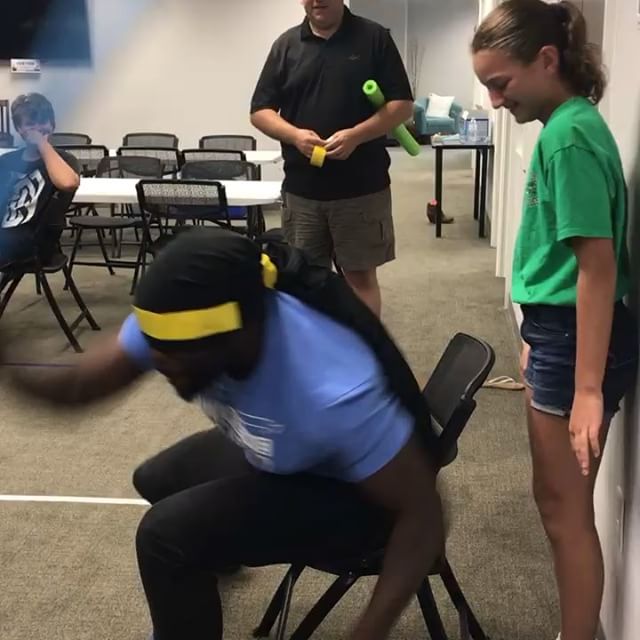In the image, set in a spacious room resembling a school or gym, an African American man sits on a black chair, seemingly in motion, as if about to jump up in surprise. He wears a blue shirt, and white, blue, and black pants. His head is covered with a black hood or do-rag, secured with yellow tape wrapped around it. Behind him, a very thin young girl in a green shirt and blue jean shorts is laughing. To the left, another child, a young woman in a black shirt with a white logo, is sitting on a folding chair in front of a white table, smiling with her hand covering her mouth. In the background, a Caucasian man dressed in a black shirt and green cargo pants holds yellow tape and a green swimming pool tube, implying he played a part in blindfolding the seated man. Surrounding them are black chairs, white tables, and in the far part of the room, a teal armchair with a white pillow, a laptop, a bottle of water, and a flat screen TV mounted on the wall. The scene captures what appears to be a playful moment among friends or participants of an activity, likely in a lively and cheerful setting.